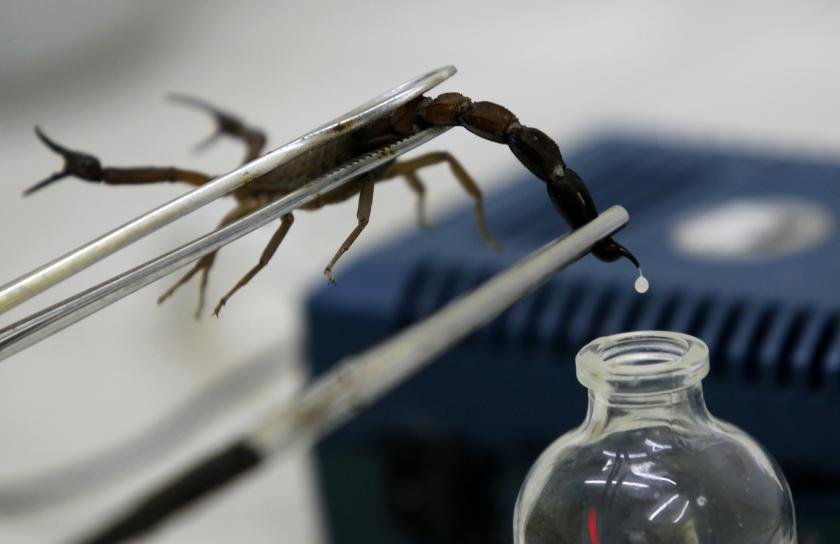In this highly detailed and realistic photograph, taken within what appears to be the blurry interior of a building or science lab, a live black scorpion is prominently featured in sharp focus against a white background. Two pairs of stainless steel tweezers are used to meticulously hold the scorpion in place: one set grips its torso, while the other set firmly squeezes its tail over a clear glass bottle positioned in the bottom right corner. The scorpion's tail bends slightly to the right, where a single white drop of venom is visibly being extracted from the stinger. The scorpion's claws face left, and its legs dangle down. In the blurred background, a blue machine or piece of equipment can be vaguely discerned, providing a subtle hint at the scientific nature of the setting.